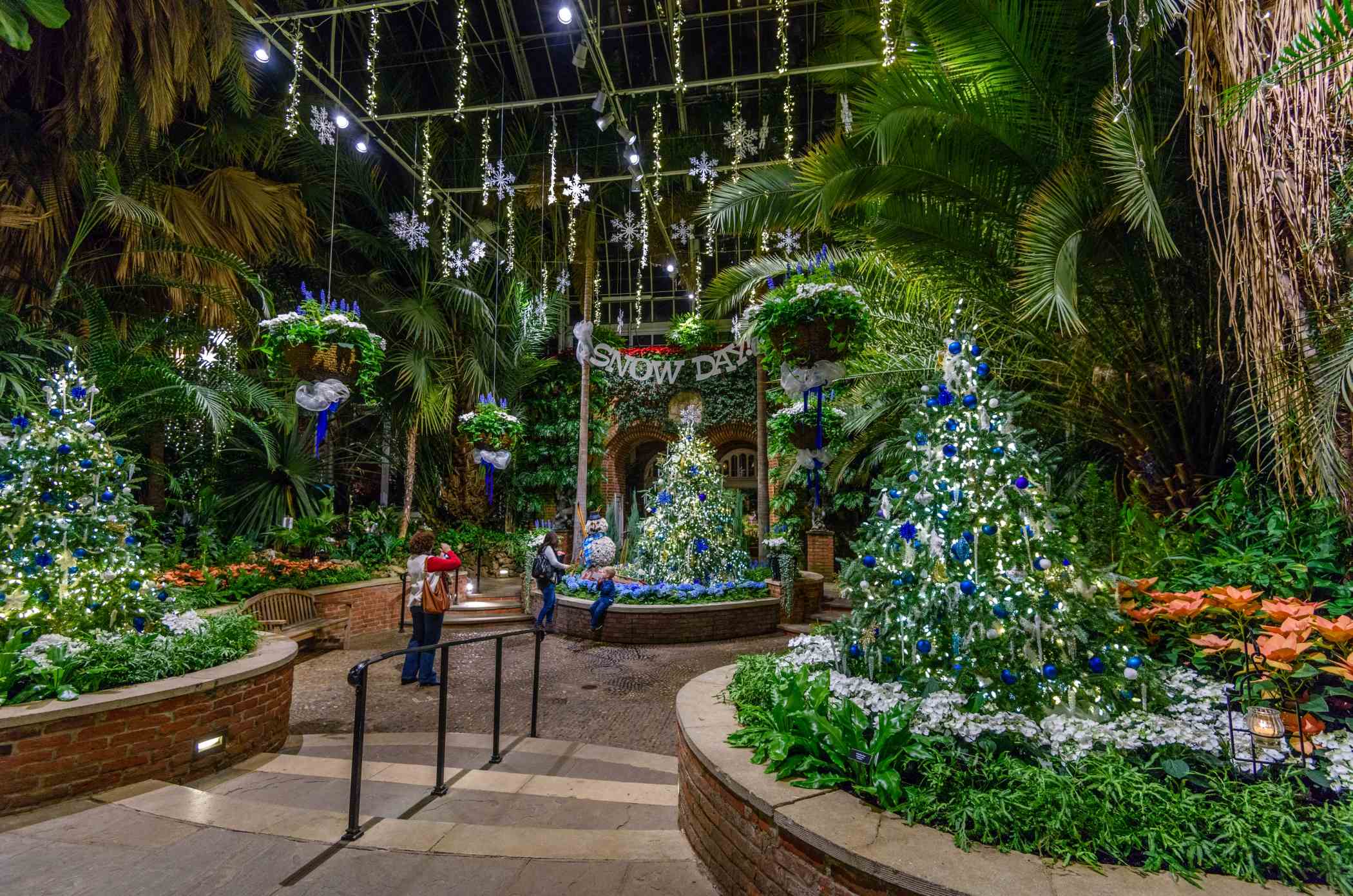This photograph captures the enchanting ambiance of an indoor botanical garden transformed with festive Christmas decor, blending tropical greenery with holiday cheer. The space features towering palm trees and lush plants interspersed with smaller triangular Christmas trees adorned in silver garland and blue glass ornaments. Positioned within raised brickwork planters, these Christmas trees frame a central walkway and staircase flanked by a metal handrail. Descending the three steps leads to another circular planter, around which stands a prominent Christmas tree, distinguished by a "Snow Day" banner above it. This central tree also boasts a snowman figure and additional blue floral decorations at its base. Stretching upwards, the lofty ceiling is supported by metal rafters, from which white decorative snowflakes and golden icicle string lights dangle, casting a festive glow. In the scene, an adult and a small child pose by the central Christmas tree, while a woman, possibly a grandmother, stands a short distance away, capturing the moment on camera.